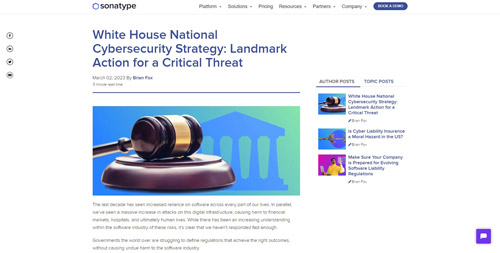A blurry screenshot from an online news article titled "White House National Cyber Security Strategy: Landmark Action for a Critical Threat" from Sonatype. The image features a blue and green box with a graphic of a judge's gavel and its base. The gavel, a dark cherry brown color with a gold band around the middle, is intricately lathed with grooves and a long handle. The wooden base appears strong and sturdy. In the green background of the box, an image of a courthouse can be discerned.